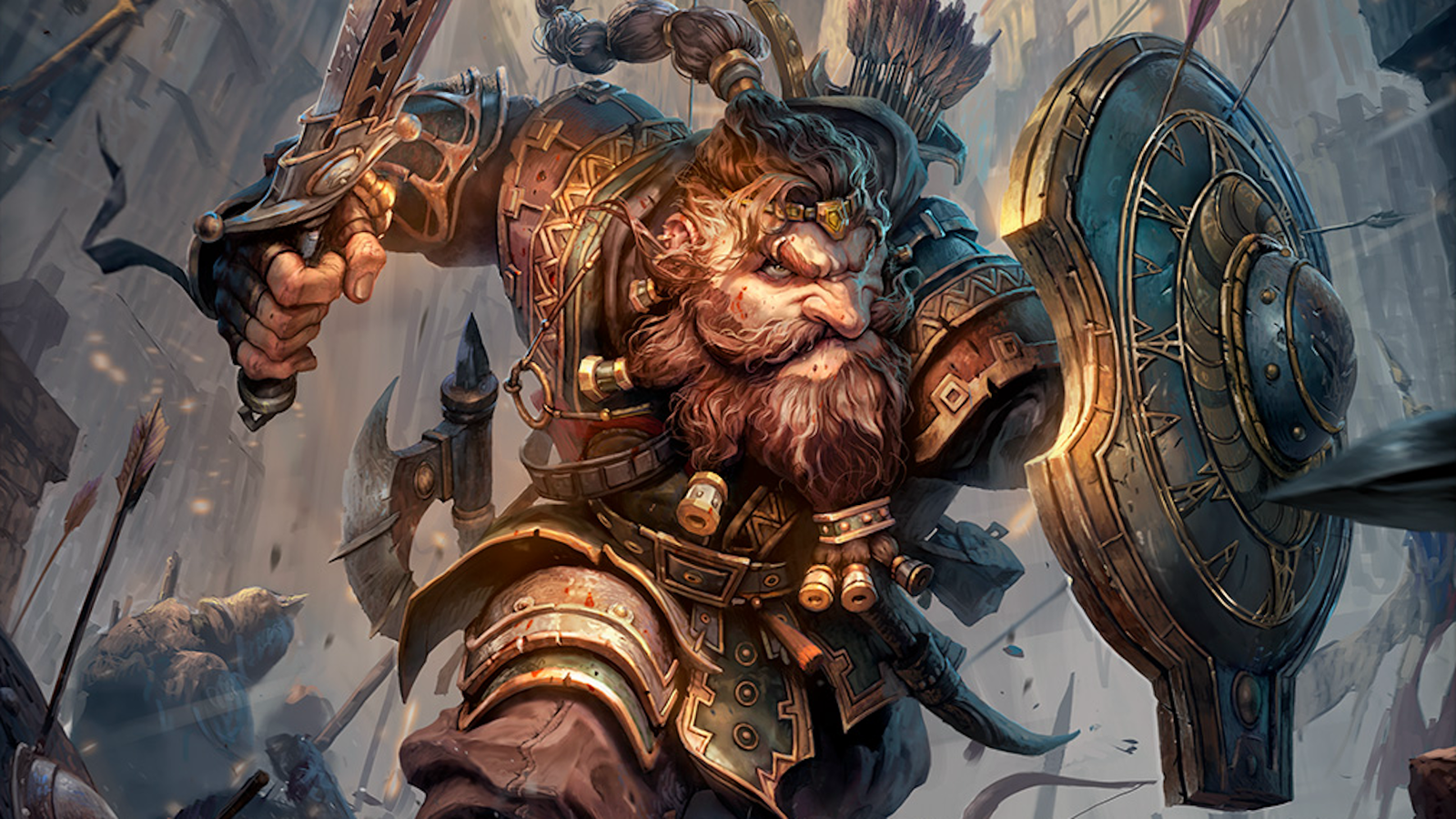The image appears to be a highly detailed, colorful illustration, possibly from a cartoon movie, animated series, comic book, or graphic computer game. It depicts a fantasy warrior, who may have a Viking-like appearance, charging into battle. He has reddish-brown hair and a long, elaborately adorned beard, with some parts decorated with gold-colored jewelry. His hair is styled in a long ponytail with sections tied off, reminiscent of certain traditional Asian hairstyles.

The warrior's expression is fierce, with large, menacing eyes and prominent eyebrows. His nose is notably big. He's clad in ornate armor with red, green, and gold detailing, and wears what look like leather pants. In his right hand, he wields a massive, intricately crafted silver sword, prepared to strike. His left arm is forward, holding an ornate, turquoise shield adorned with gold trim and decorations, which is already embedded with several arrows, implying he's been under heavy attack. The shield has a thick, metal-like construction.

In the chaotic background, arrows are flying through the air, striking various targets, and the scene has a grim atmosphere with fallen warriors and smoke, embodying the din of battle. An additional battle axe can be seen on his side, and a quiver of arrows is visible behind him, further emphasizing his readiness for combat.